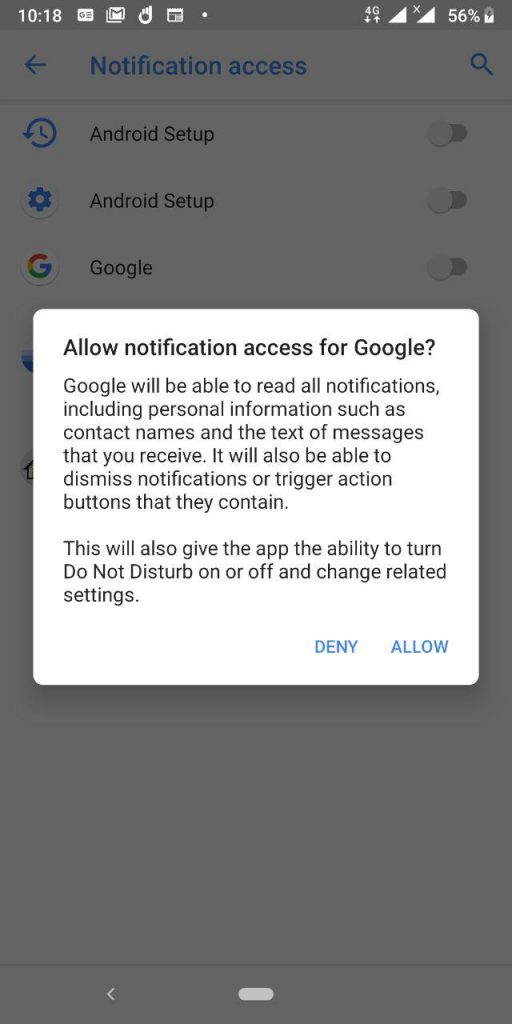This is a detailed screenshot of a phone interface. The background of the screenshot is a muted gray. At the top left corner, the time displays as 10:18 AM in white font, alongside various status icons. On the right side of the status bar, the screen indicates a 4G network connection with full signal strength (four bars) and a battery life at 56%.

The notification panel is expanded, revealing notifications and settings in a slightly dimmed overlay. At the top, a notification with "Notification access" in bold blue letters is visible. Below this, the words "Android Setup" are repeated twice with distinctive icons next to each entry: a clock icon to the right of the first "Android Setup," and a gear icon to the left of the second "Android Setup." Following these, the word "Google" is listed, preceded by the colorful Google logo.

Dominating the center of the screen is a prominent white dialogue box with black text. The message in the white box informs the user that they need to allow notification access for Google. It explains that Google will gain the ability to read all notifications, including personal information such as contact names and the texts of received messages. Further, Google will be able to dismiss notifications or trigger associated action buttons. The bottom part of the message elaborates that this permission will also allow Google to control the "Do Not Disturb" mode and modify related settings.

At the bottom right corner of this dialogue box, there are two interactive buttons labeled "Deny" and "Allow" in blue letters, inviting the user to make a selection.